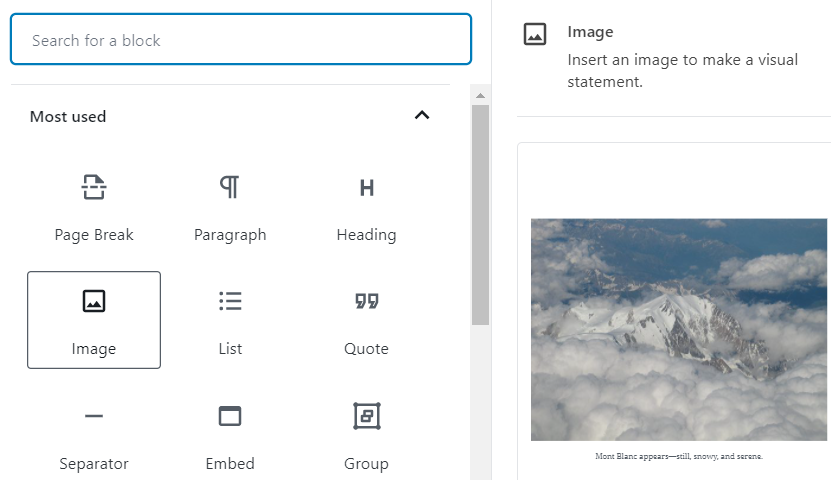Screenshot Description:

The image is a screenshot displaying a user interface for inserting content blocks. The interface consists of two primary sections arranged vertically, taking up roughly two-thirds (left section) and one-third (right section) of the screen, on a predominantly white background.

In the left section, at the top left corner, there is a blue-outlined rectangular box labeled "Search for a block." Directly below this search box, there is a vertical scroll bar on the right side of the left section, indicating more content can be displayed.

This left section lists several commonly used blocks under a header labeled "Most Used," organized into rows:
- **First Row:** Icons for "Page Break," "Paragraph," and "Heading."
- **Second Row:** Icons for "Image," "List," and "Quote."
- **Third Row:** Icons for "Separator," "Embed," and "Group."

The scroll bar suggests that additional blocks can be accessed by scrolling.

In the right section, the top part displays a small, blank image icon featuring two stylized mountains, accompanied by the label "Image" and the text "Insert an image to make a visual statement." 

Below this placeholder is a photograph captioned "Mont Blanc appears still snowy and serene," showing an image of Mont Blanc, emphasizing its snowy and tranquil appearance.

Overall, the screenshot depicts a content management interface where the user is in the process of inserting an image block with a layout designed for user-friendly navigation and insertion of various content types.